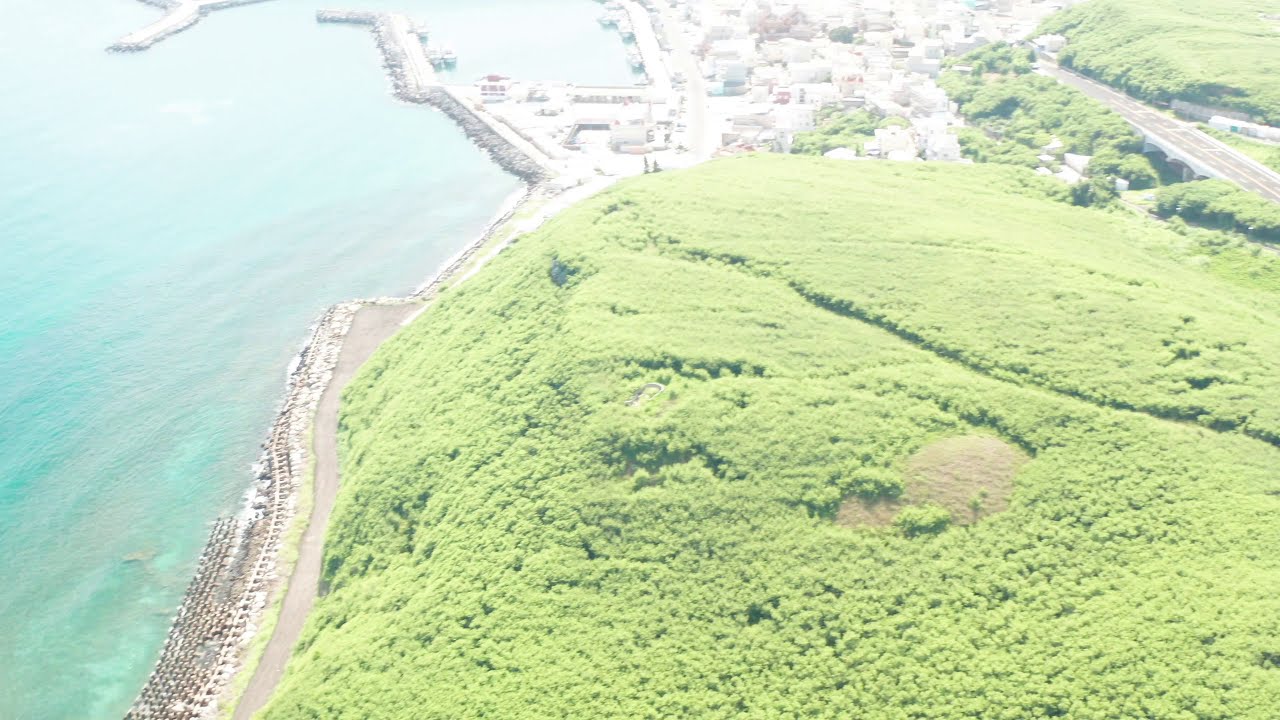This aerial drone shot captures a sprawling beach town city from a significant height, revealing a sun-drenched landscape with washed-out colors due to the overexposure. Dominating approximately 60% of the lower right portion of the image is a verdant expanse of bright lime-green trees, grass, and bushes, hinting at a hill or gently sloping terrain. The vibrant greenery contrasts starkly with the rest of the landscape, which is bathed in a glaring white light, lending the photo a hazy, almost ethereal quality.

To the left of the grassy area, cliffs drop down to meet a striking turquoise ocean that spans the left edge of the image. Though the water is visible, the glare obscures the finer details, making the color appear almost sky blue. Scattered asymmetrically across the upper half of the photo, small, nondescript buildings dot the landscape, creating a patchwork of what seems to be a distant town. The indistinct quality of the structures suggests numerous houses or other buildings, but their small size and the lack of clarity make them difficult to identify precisely.

A dark roadway can be seen threading through the upper right corner, running parallel to a marina that sits at the top center of the image. Docks are faintly visible, though potential boats are lost in the photographic overexposure. Additional roads meander through the image, appearing sporadically across the landscape, further emphasizing the man-made aspects amidst the natural setting. All these elements culminate in a scenic yet somewhat surreal depiction of a lush, coastal town under a bright, overwhelming sun.